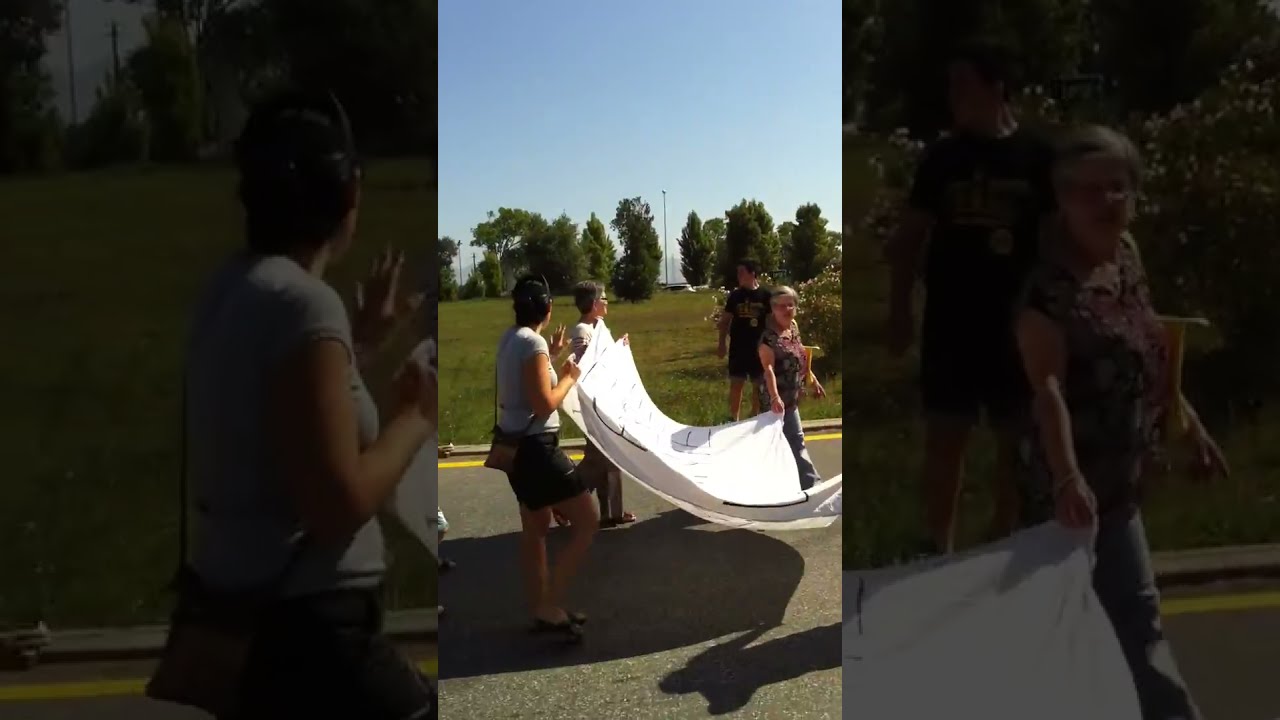In this outdoor photograph, four people are walking along a wide, paved road. On the left, a man in a red shirt holds the hand of a little girl dressed in light-colored shorts and a shirt; she clutches a long, indistinct object. On the right, two women are visible; one has a long ponytail and is dressed in a white t-shirt and shorts, holding a hand-painted white banner with pink lettering. The second woman’s presence is hinted by the darkness ahead of the banner-holder. Their shadows stretch behind them, suggesting that the photo was taken either mid-morning or mid-afternoon under a clear blue sky. Behind the group, an expansive, grassy field is dotted with pink or red flowers, bordered by orange temporary fencing. Further back, there are several buildings and a towering electrical structure with power lines, and a hill can be spotted on the far right.